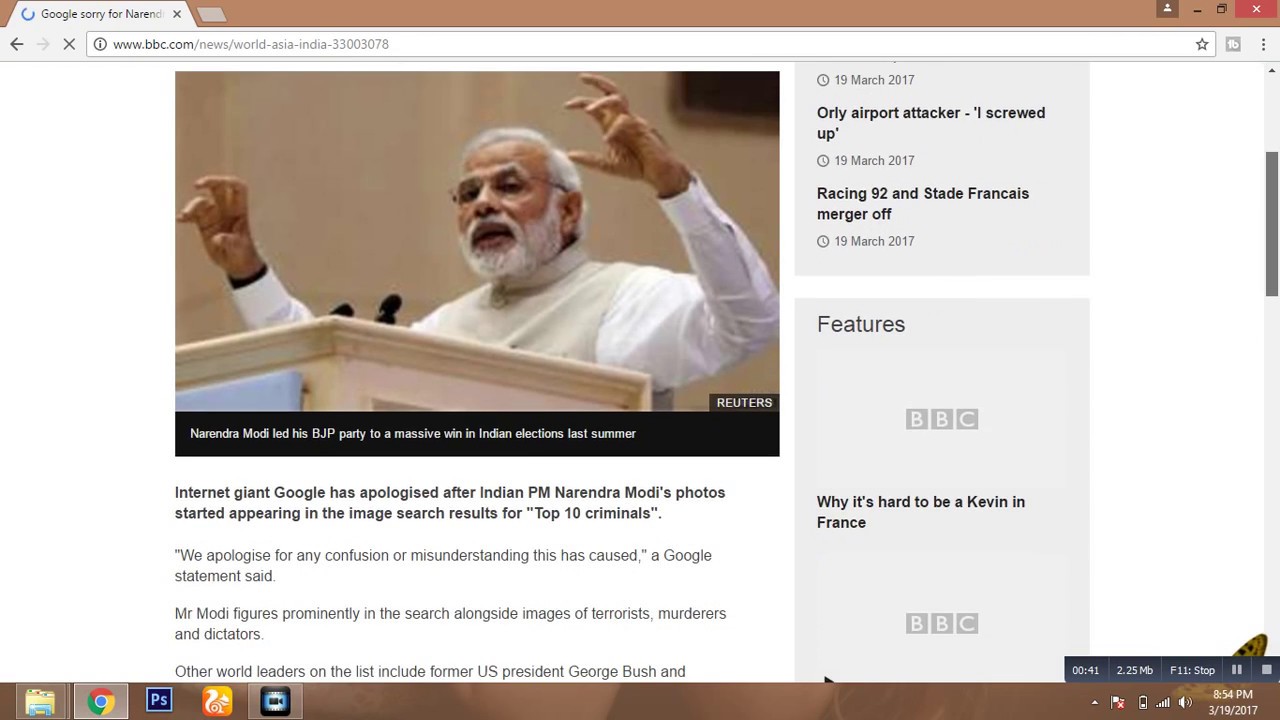This screenshot captures a detailed view of a computer desktop. The desktop features an internet browser window open, specifically displaying the search results from the website bbc.com. The URL in the address bar reads "www.bbc.com/news/world-asia-india-33003078." The web page focuses on a headline story about Indian Prime Minister Narendra Modi.

The main visual content of the browser window shows a prominently placed image of Narendra Modi, credited to Reuters. In the image, Modi is clad in a white top and glasses, standing at a podium with both hands raised mid-speech. His expression appears earnest and engaged.

The article headline reads, "Narendra Modi led his BJP party to a massive win in Indian elections last summer." The story further explains that "Internet giant Google has apologized after Indian PM Narendra Modi's photos started appearing in the image search results for 'top 10 criminals.' 'We apologize for any confusion or misunderstanding this has caused,' a Google statement said." The narrative mentions that Modi's image was displayed alongside those of terrorists, murderers, and dictators. The text also notes that other world leaders featured in the list included former US President George Bush, though the sentence is cut off before it completes.

The bottom part of the screenshot showcases the typical menu bar of the computer's operating system, indicating the various applications and functions open or available for access at the time.